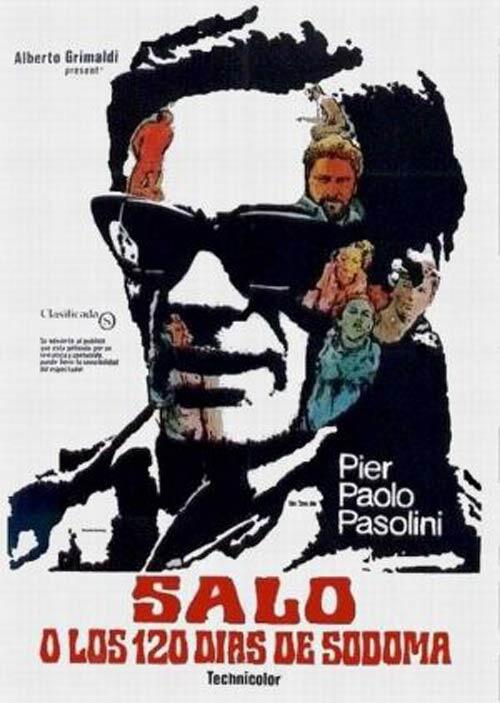This image is a detailed and artistic poster, likely for a movie or play, featuring a stylized black-and-white drawing of a man's head and bust. The man, who appears to be slightly older, is wearing sunglasses and is depicted from the shoulders up against a white background. His face encompasses various colorful, smaller illustrations, including several human figures engaged in different activities—one wearing blue, another in red, and another in orange—all positioned particularly around the left side of his face. The text "Alberto Grimaldi presents" is displayed in a new Roman font on the top left, showcasing the producer. Beneath the man's head, in white text, the actor "Pier Paolo Pasolini" is credited, followed by the title "Salo, O los 120 Días de Sodoma" in red letters at the bottom, highlighting the controversial film's name. Additional small, unreadable text is also present on the left side. The poster is bold and visually striking, combining monochrome elements with vivid color illustrations, making it a captivating advertisement.